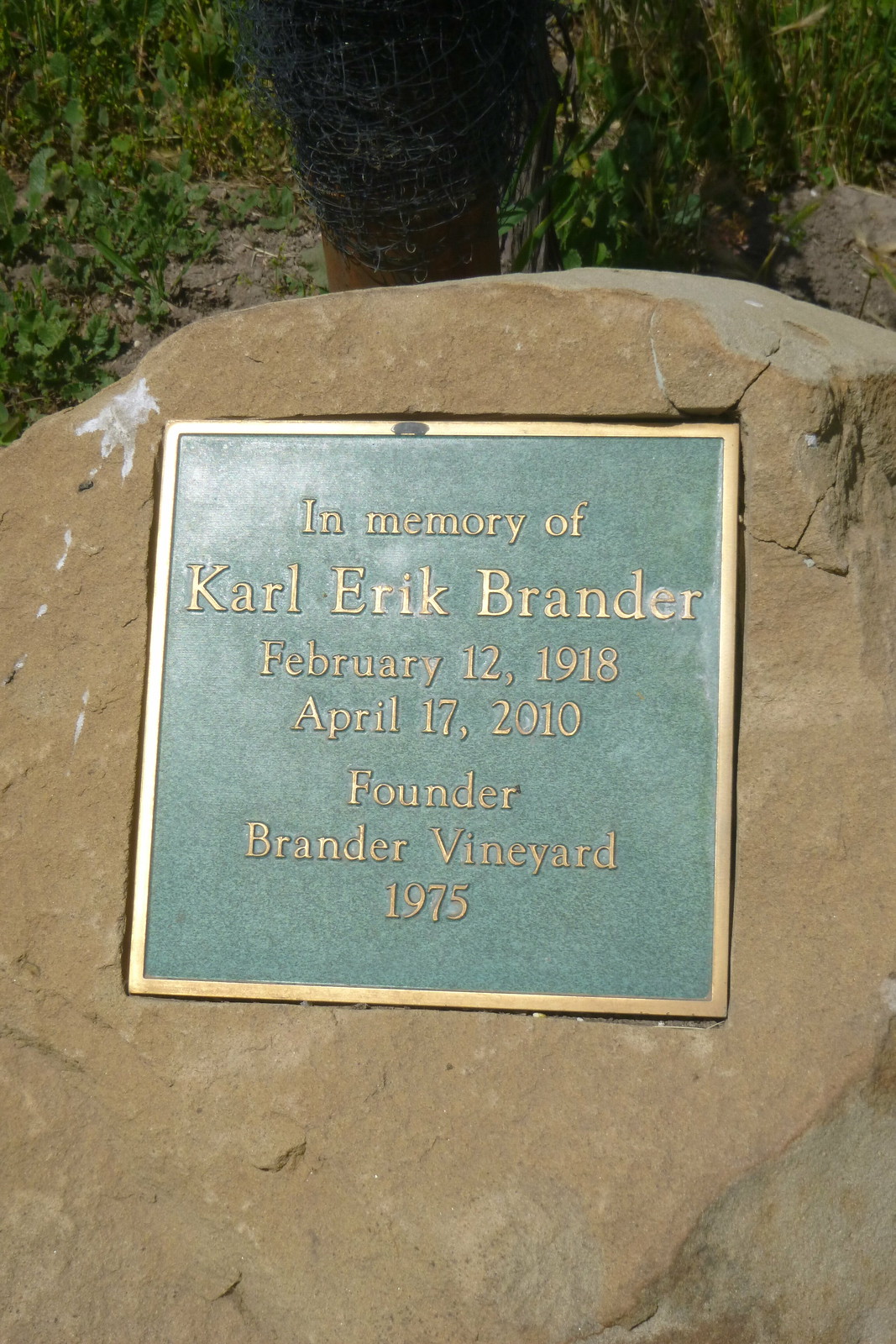In the image, there is a large tan boulder set outdoors, with a square-shaped memorial plaque embedded into its surface. The boulder, which is predominantly light gray with hints of tan, features minor cracks around its upper right side and has a splatter of bird droppings on its upper left. The sun highlights the upper left-hand corner of the boulder, adding a subtle glow. The plaque, which appears to be made of a blue-green stone, has a gold or bronzish-gold border and matching gold text. The inscription reads, "In memory of Carl Eric Brander, February 12, 1918 to April 17, 2010. Founder, Brander Vineyard, 1975." Behind the boulder, some vegetation, including a tree trunk, small bushes, and blades of grass, can be seen, providing a natural and serene backdrop.